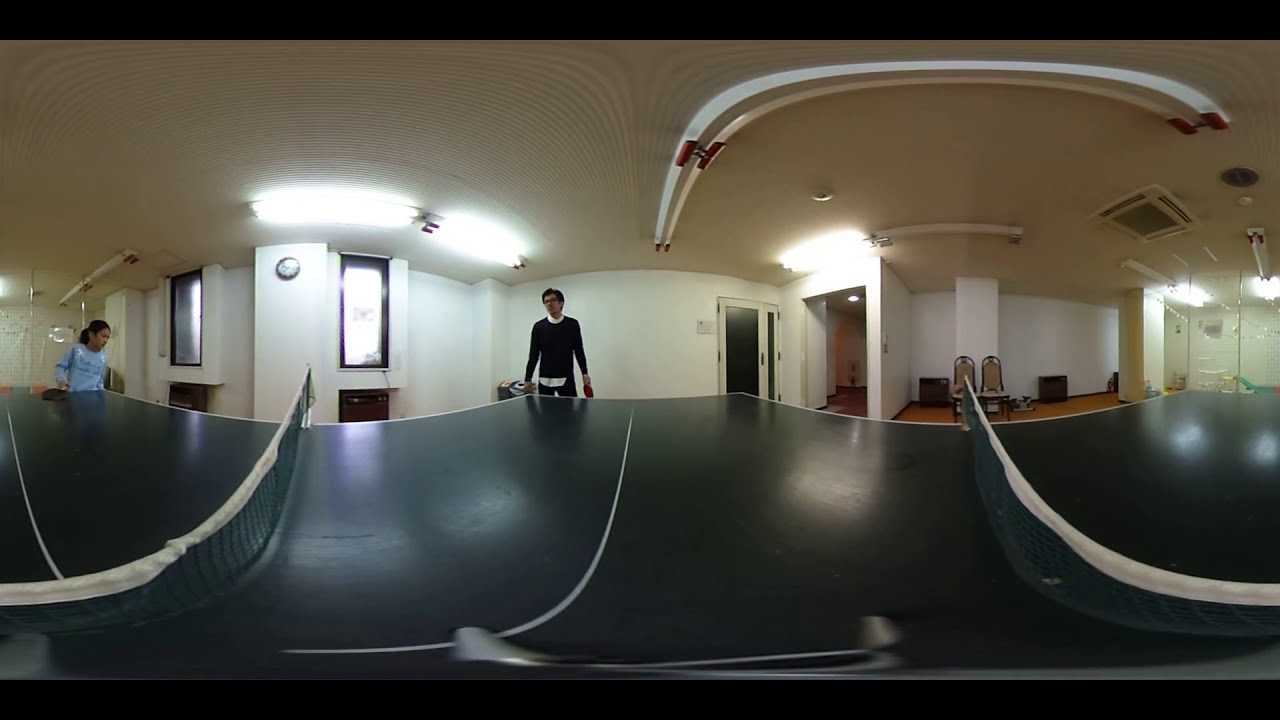The image captures a 360-degree, VR-distorted view of a recreational facility, specifically featuring a ping-pong table. The elongated, warped view reveals various elements: to the left, a girl in a light blue top is holding something, while to the right, a boy in a black shirt stands near the table. The ping-pong table itself is dark blue, with a net stretching across it that seemingly bends due to the lens distortion. Bright, fluorescent overhead lights appear warped, contributing to the surreal, science-fiction-like ambiance. The room includes glass doors and windows that frame the space, which also encompasses a small waiting area with chairs, suggesting it could be a multipurpose rec center. The storage shed atop the image, combined with the extreme lens distortion, creates an intriguing, almost disorienting perspective that blurs conventional spatial boundaries.